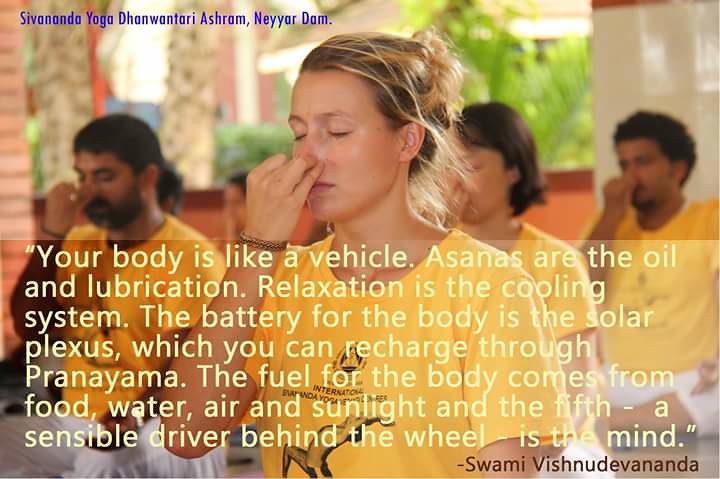The image depicts a diverse group of individuals participating in a yoga or meditation class, seated together on the ground in a tranquil indoor setting. Most of them appear to be in the middle of practicing a breathing exercise, with their fingers placed on their noses and their eyes gently closed. All participants are dressed uniformly in short-sleeved yellow shirts, and some also in white shorts. Framing the scene, the building's open layout allows a glimpse of lush greenery outside, including palm trees and large ferns, suggesting a serene, natural environment.

Positioned above the group, blue text reads "Sivananda Yoga Dhanwantari Ashram, Nair Dam." Central to the image, prominently displayed in a slightly white box, is an enlightening quote from Swami Vishnudevananda: "Your body is like a vehicle. Asanas are the oil and lubrication. Relaxation is the cooling system. The battery for the body is the solar plexus, which you can recharge through pranayama. The fuel for the body comes from food, water, air, and sunlight. And the fifth, a sensible driver behind the wheel is the mind." The quote emphasizes a holistic view of bodily health and the importance of yoga practices.